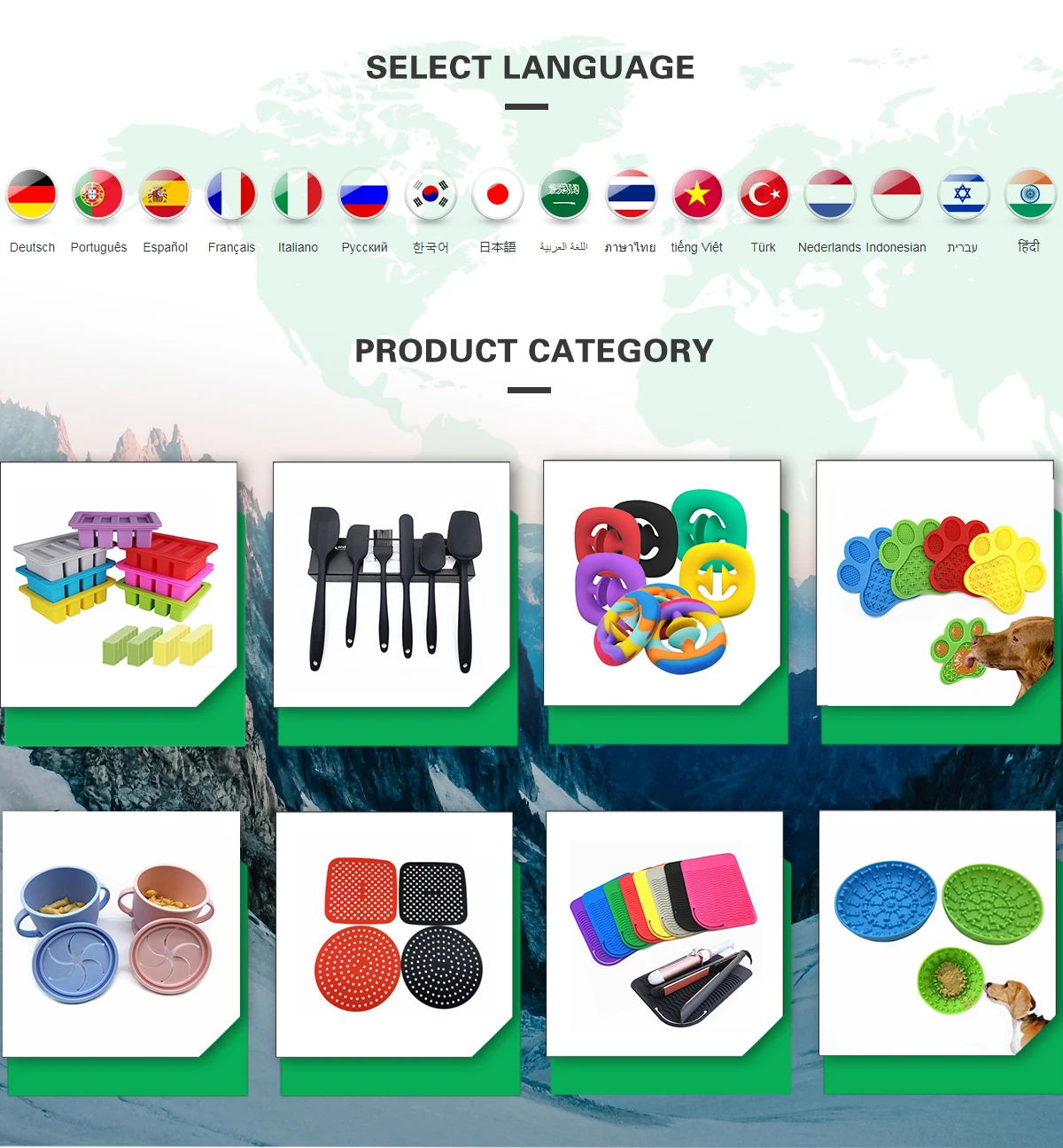The image showcases a colorful array of plastic items, seemingly targeted at either children or dogs. The items include ice cube trays, spatulas, vibrant rings, and miniature dog paw-shaped objects. There are also images of dogs interacting with some of these items, suggesting they might be chew toys. Among these, there are also confusing additions like a pot with a lid and what appear to be medical instruments, which don't clearly indicate their purpose or appeal to dogs. At the top of the image, there is a “Select Language” option that offers a wide range of languages, including German and Farsi, indicating a global reach. The overall scene is perplexing as it is unclear exactly who these products are intended for.